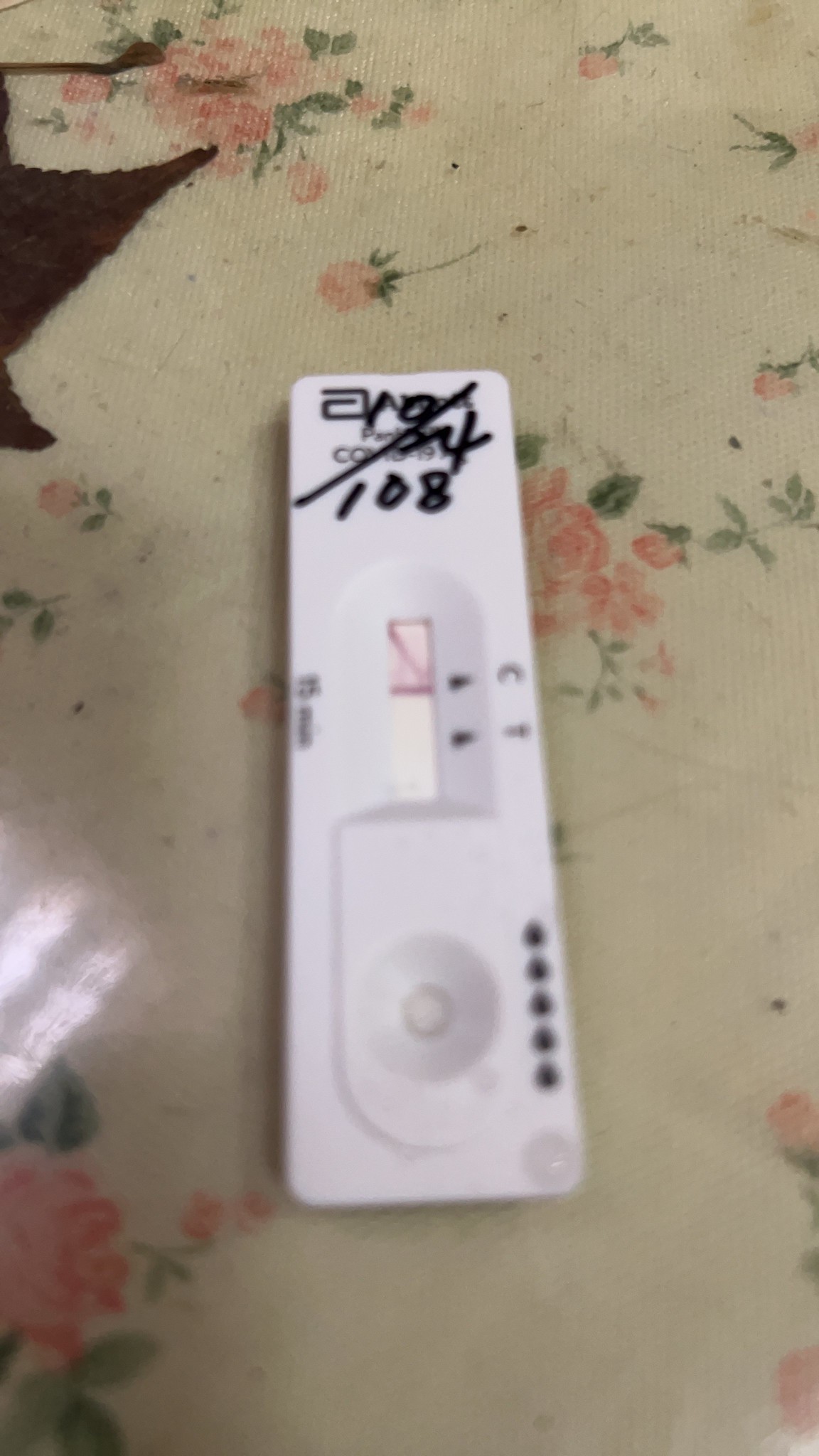This image features a somewhat blurry COVID-19 test kit placed on a surface that appears to be a dirty tablecloth. The test kit itself is a rectangular, white object with distinctive markings and components. At the top section, there is a circular indentation housing a test pad. Adjacent to this circle, along the right side, are a series of black dots. Further down, the second section of the test kit displays the letters "C" and "T." In this particular test, the "C" line is solid, indicating the control line, and there is a shaded pink line suggesting test results. 

At the bottom end of the test kit, the text "COVID-19" is visible, though it has been crossed out with a diagonal black marker line. Below this, the number "4" is printed, and above the marker line, some additional text is present. The number "108" is handwritten underneath the crossed-out area. The test kit rests on a tablecloth that appears soiled. Beside it, there is a star-shaped crocheted item with multiple points, featuring pink flowers and green leaves.